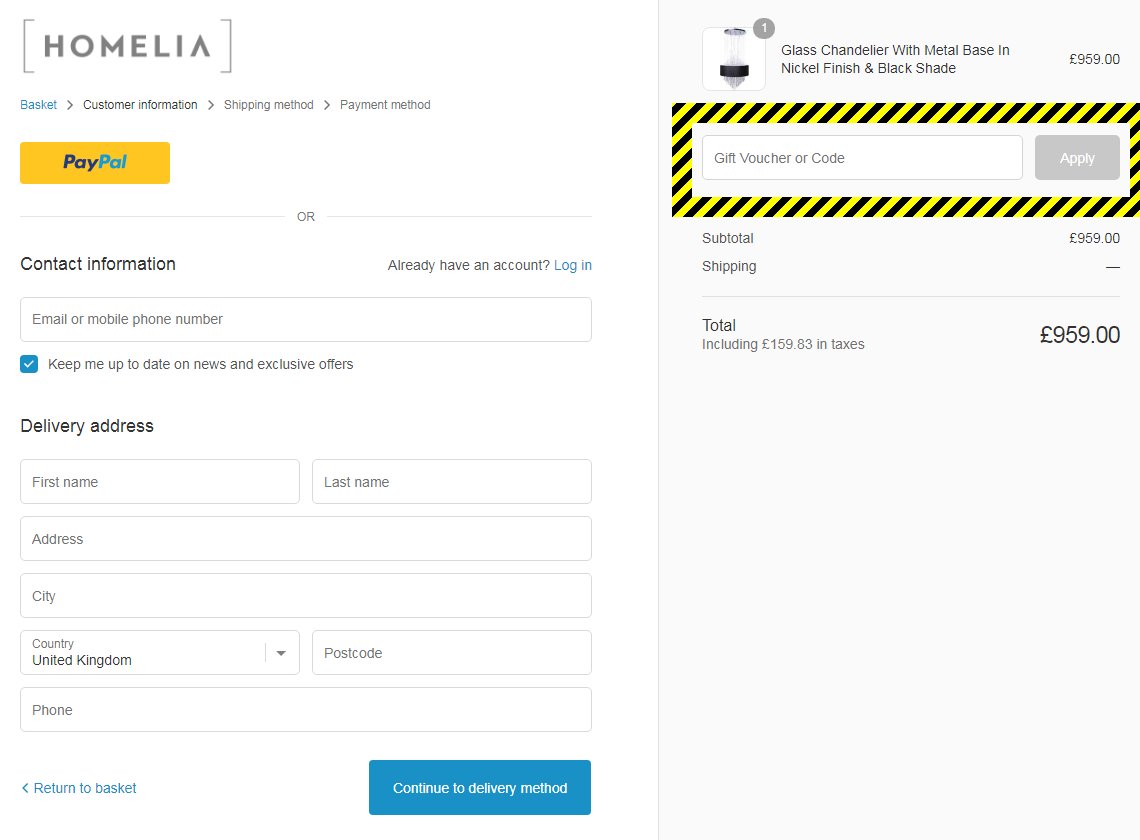The image depicts a webpage from the online store "Homelia." At the top of the page, there are navigation checkpoints labeled "Basket," "Customer Information," "Shipping Method," and "Payment Method," each accompanied by forward arrows. Below these checkpoints, there is a prominent yellow PayPal button. An "or" separator follows, leading to fields requesting contact information. A prompt invites users who already have an account to log in using a prominently blue "login" link.

The contact information section includes a field for an email or mobile phone number and a checkbox to opt-in for updates on news and exclusive offers. Further below, there is a delivery address section requesting first name, last name, address, city, country (pre-selected to United Kingdom), postcode, and phone number.

At the bottom of this section, there are two blue buttons: one labeled "Return to Basket" and the other "Continue to Delivery Method."

The next part of the page displays details of the item being purchased: a large glass chandelier with a metal base, a nickel finish, and a black shade. The chandelier, which appears mostly silver with a black base shade at the bottom, is priced at £959.00. Next to the chandelier's information, there is a form field for entering a gift voucher or promotional code, bordered in yellow and black, along with an "apply" button. The subtotal is listed as £959.00, with shipping costs marked by a line, indicating no additional charge. The total price, including taxes of £159.83, is summarized at £959.00.